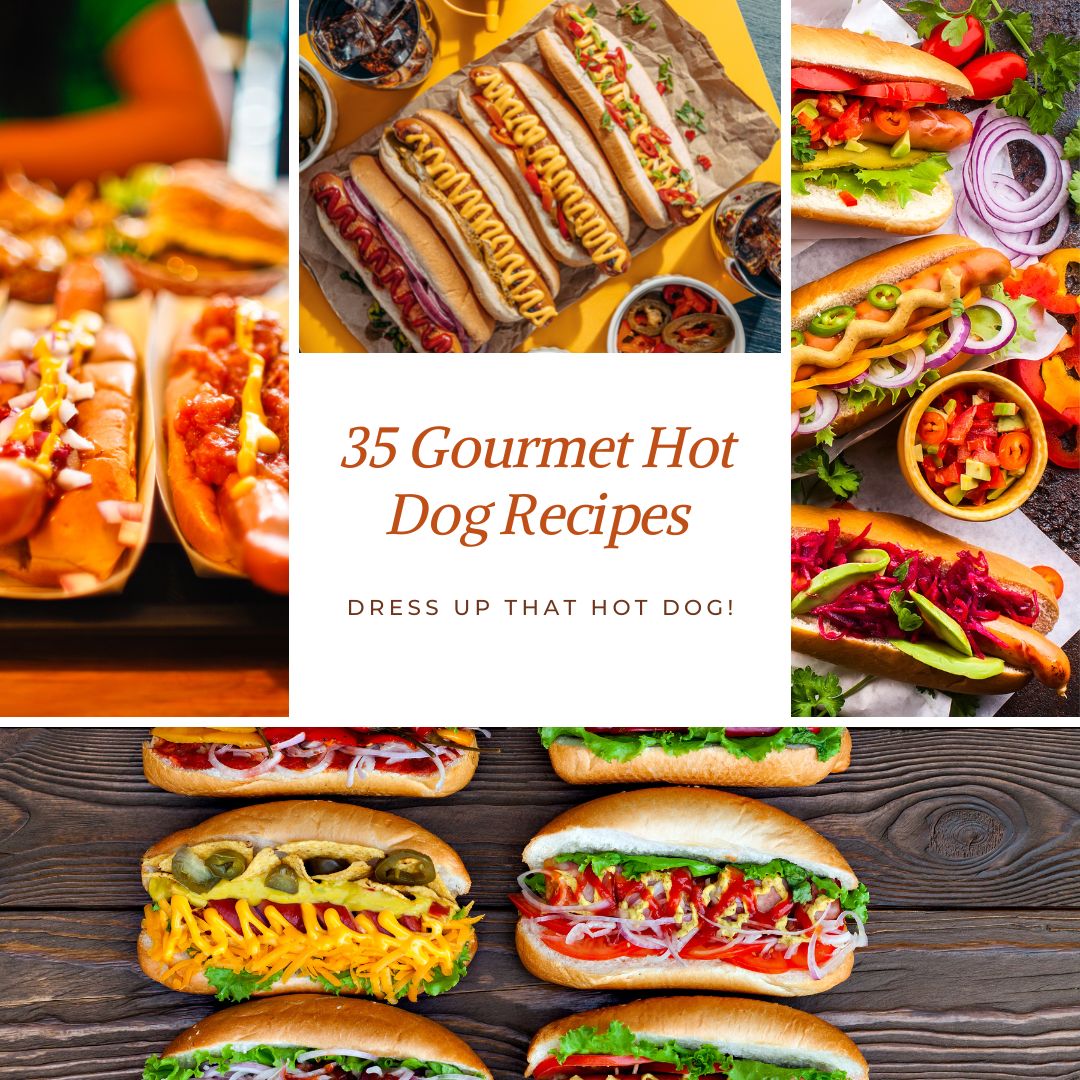This image looks like a promotional cover for a cookbook or a blog post, showcasing a collage of various gourmet hot dog recipes. At the center of the image, inside a white text box with brown-orange font, it reads, "35 Gourmet Hot Dog Recipes. Dress up that hot dog." Surrounding this central text box are four distinct images, each displaying different hot dog arrangements with a variety of toppings.

On the left, there's an image featuring a chili cheese dog with cheese sauce, mustard, and another one with ketchup and chopped onions in to-go containers. Above the central text box, a row of four hot dogs shows diverse toppings: one with ketchup, two with mustard, and another with a combination of bacon or peppers and mustard. 

To the right, the bottom images display more specialty hot dogs. Various options include toppings like peppers, red onions, jalapenos, cheese, lettuce, and avocado, adding vibrant colors and flavors to each hot dog. The collage provides an enticing visual that invites the viewer to explore the creative and gourmet possibilities for dressing up a classic hot dog.